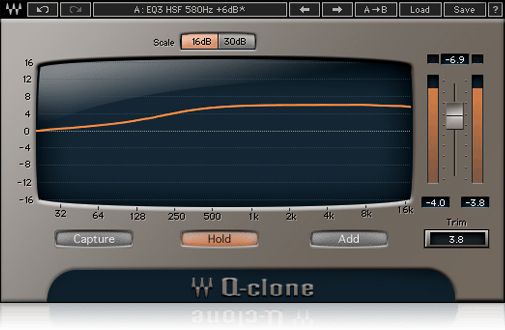The image depicts a complex gray electrical panel with a black border at the top. In the far left corner, there's a 'W' next to a button with an arrow that circles and then points down to the left. Adjacent to this is another arrow in a square moving down and to the right. Following these arrows is a prominently outlined white bar labeled "AEQ3HSF580HZ6DB", suggesting it could relate to sound or frequency settings. To the right, a series of buttons exist: one with a left-pointing arrow, another with a right-pointing arrow, an "A to B" button, and buttons labeled "Load", "Save", and a gray question mark.

In the center of the panel, a blue screen displays a graphical readout with blue horizontal lines and an orange ascending line from left to right. Two vertical orange bars with sliders flank the right side of the screen, with numerical values detailed at the top and bottom of these bars. Beneath the screen sit several buttons: starting from the left, there's an orange button marked "Scale 16 dB", a gray button marked "30 dB", a section labeled "Capture", an orange button "Hold", and further right, a black button marked "Trim".

Further below, four additional buttons are displayed on the bottom border, with the labels "W", "Q", and "Q-clone" in silver lettering. The screen appears to illustrate a frequency readout with the y-axis ranging from 16 dB at the top to -16 dB at the bottom, and an x-axis ranging from 32 to 16 K, indicating this panel measures or manipulates audio frequencies.